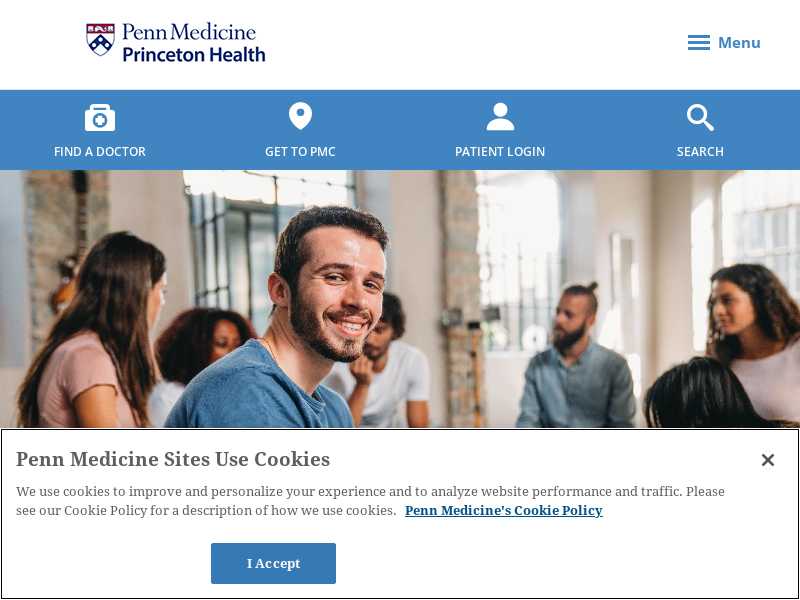In this image, we observe the homepage of Princeton Health's website, specifically focused on their pain medicine department. Prominent navigation categories include "Find a Doctor," "Get to PMC," "Patient Login," and "Search." The site also informs visitors about its use of cookies to enhance user experience and analyze web traffic, with links to their detailed Cookie Policy and a button for users to accept the policy. The page features a header image showcasing six individuals—three males and three females—likely representing the diverse team of medical professionals dedicated to providing pain management care.